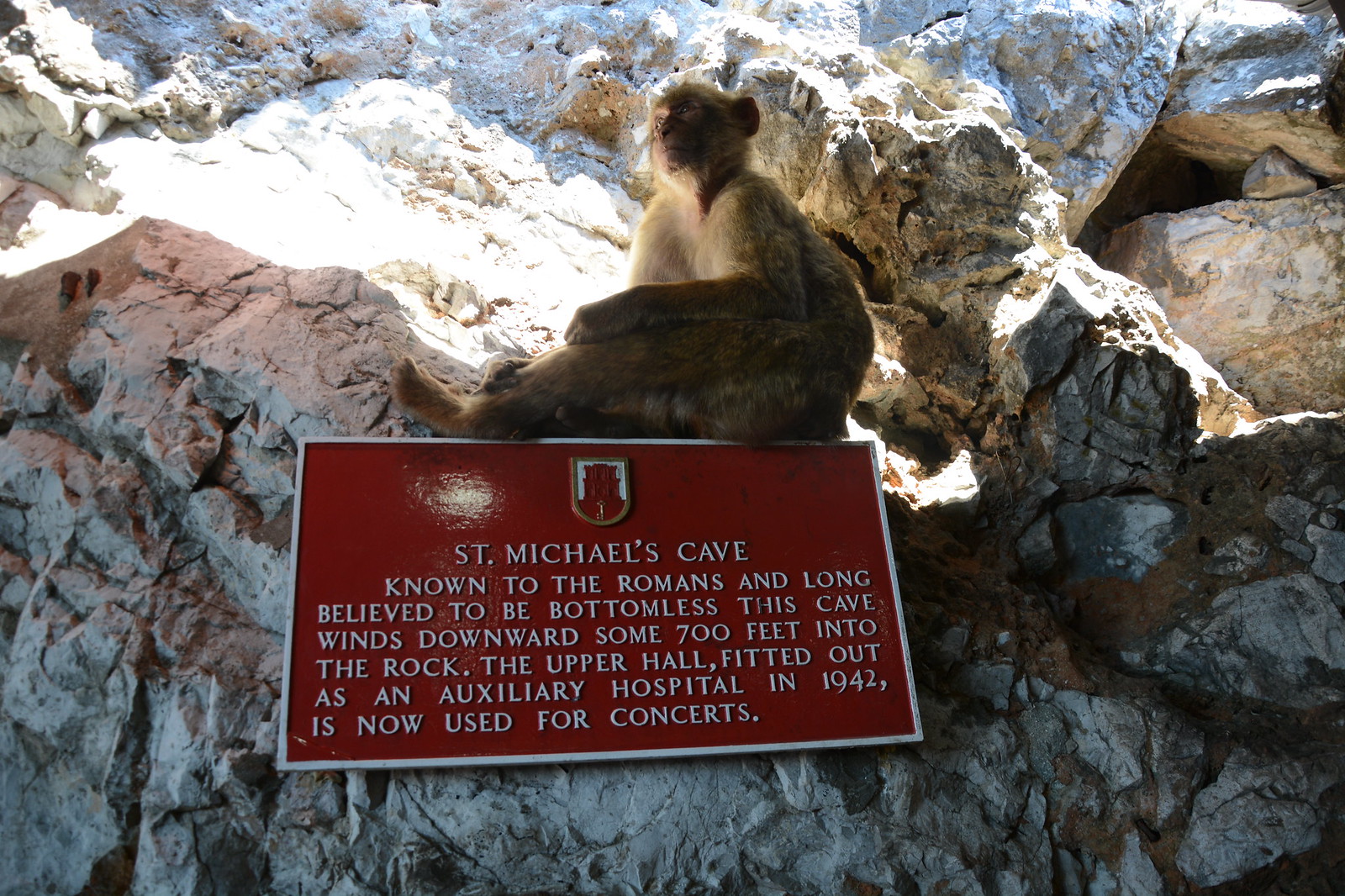The image depicts a rock wall constructed with gray boulders, upon which a red plaque with white text has been mounted. The plaque reads: "St. Michael's Cave, known to the Romans and long believed to be bottomless. This cave winds downward some 700 feet into the rock. The upper hall, fitted out as an auxiliary hospital in 1942, is now used for concerts." Perched atop the plaque is a large brown monkey, approximately the size of a toddler, boasting a white chest. The monkey is seated with his paws on his legs, gazing off into the distance to the left. Sunlight backlights the scene, indicating the area around the cave is not entirely enclosed.